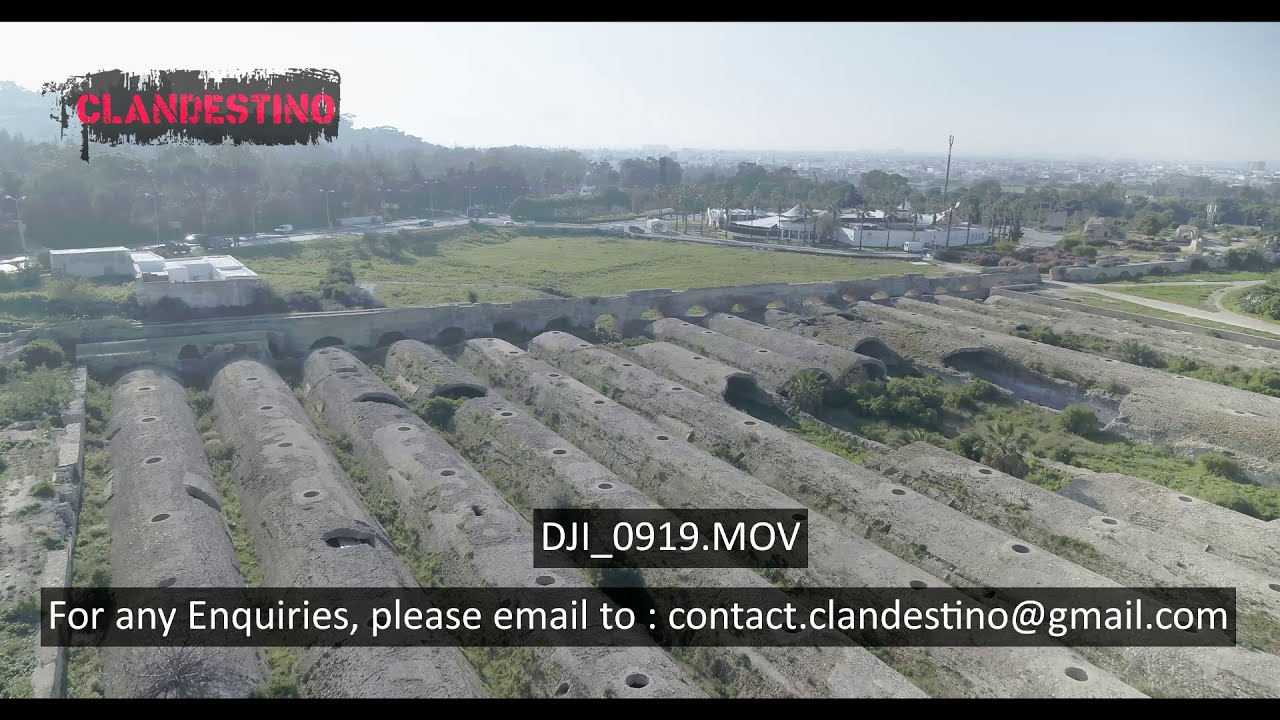The image is an outdoor scene captured in what appears to be the middle of the day, showing a varied landscape of both natural and man-made structures. Dominating the lower half of the image are numerous old stone or concrete tunnels and pylons, some of which are broken or partially collapsed, displaying curves and circular holes running across the tops. In the center of these structures, a few trees have emerged, adding natural greenery to the otherwise gray and stony setting.

Towards the middle and extending to the top of the image, the scene transitions into lush grasslands and sporadic trees, framed by various buildings to the left and right. The sky above is primarily gray, casting a muted tone over the entire photograph.

Text overlays adorn the image, with "Clandestino" written in red font with black etchings behind it in the top left corner, and "DJI_0919.mov" displayed in white font on a black box at the bottom, followed by a contact email address: "for any inquiries please email to contact.clandestino@gmail.com". The overall color palette includes shades of black, white, gray, green, and red.